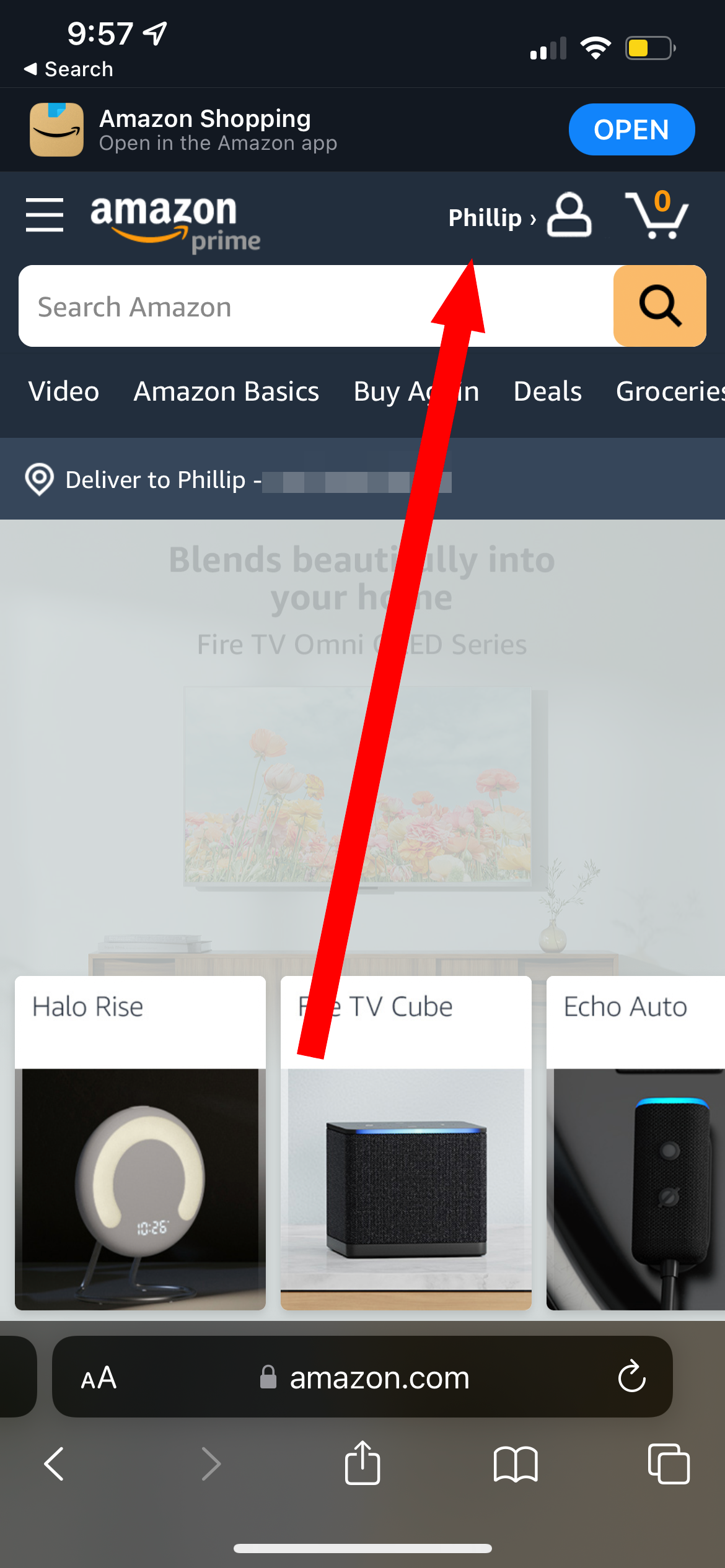### Detailed Caption for the Screenshot:

The image is a screenshot taken from a smartphone, featuring the Amazon Shopping app interface. 

- **Top Corners:**
  - On the top left corner, a white arrow is visible, likely indicating a back button.
  - The top right corner displays several status icons: a data signal, a Wi-Fi symbol, and a yellow battery icon.

- **App Header:**
  - The app header shows the text "Amazon Shopping."
  - There's an invitation to "Open in the Amazon app" with an additional prompt "Open Amazon Prime" accompanied by a red arrow pointing towards it.

- **User Interface Elements:**
  - A profile icon and a shopping cart icon (showing "0" items) are located beside the open prompts.
  
- **Search and Categories:**
  - A search bar labeled "Search Amazon" is prominently displayed.
  - Below the search bar, various shopping categories and offers are listed: "Video," "Amazon Basics," "Buy Again," "Deals," "Groceries," and "Delivery to [blurred out name]."

- **Featured Products:**
  - Various product names are mentioned, such as "Blends Beauty," "Fire TV," "Halo Rise," with accompanying images:
    - A picture of a black electronic device labeled "TV Cube."
    - Another item called "Echo Auto," depicted with a black and blue electronic device.

- **Bottom Bar:**
  - At the bottom of the screen, a black navigation bar includes symbols:
    - A small and a large letter "A" indicating text size adjustment.
    - A padlock symbol with the text "amazon.com."
    - Refresh, back, and forward arrows (the forward arrow is grayed out).
    - A white square with an upward-pointing arrow (likely a share button).
    - A book icon, a silhouette, and two overlapping squares.
    
- **Bottom Bar Background:**
  - The bar rests on a white background with a grey gradient towards the bottom.

Overall, the screenshot encapsulates a typical user experience on the Amazon Shopping app, highlighting various navigational and interactive elements.